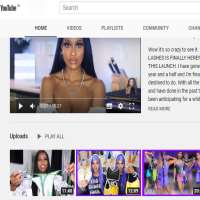This image is a screenshot of what appears to be a YouTube channel's main page. In the upper left-hand corner of the screen, there is a slightly faded YouTube logo. To the right of this logo, there's a search field typical of YouTube's interface.

Directly below the search field, there’s a playable video thumbnail featuring a woman. Above this video thumbnail, a series of menu options are visible: "Home," "Videos," "Playlists," and "Community," with a fifth option partially cut off and unreadable.

The playable video thumbnail is located on the left side, and alongside it on the right, there’s some text which is presumably a description of the video, though it is too blurred to decipher.

Beneath this section, there is a category labeled "Uploads," accompanied by a "Play All" button. Three individual video thumbnails are displayed below, indicating videos that the channel owner has uploaded.

The entire page features a white background with dark black font, maintaining a clean but unremarkable aesthetic. The visual elements of the videos themselves are not in color, contrary to typical YouTube video thumbnails. Overall, the image captures the fundamental layout and elements of a standard YouTube channel page, although some text details remain unclear.